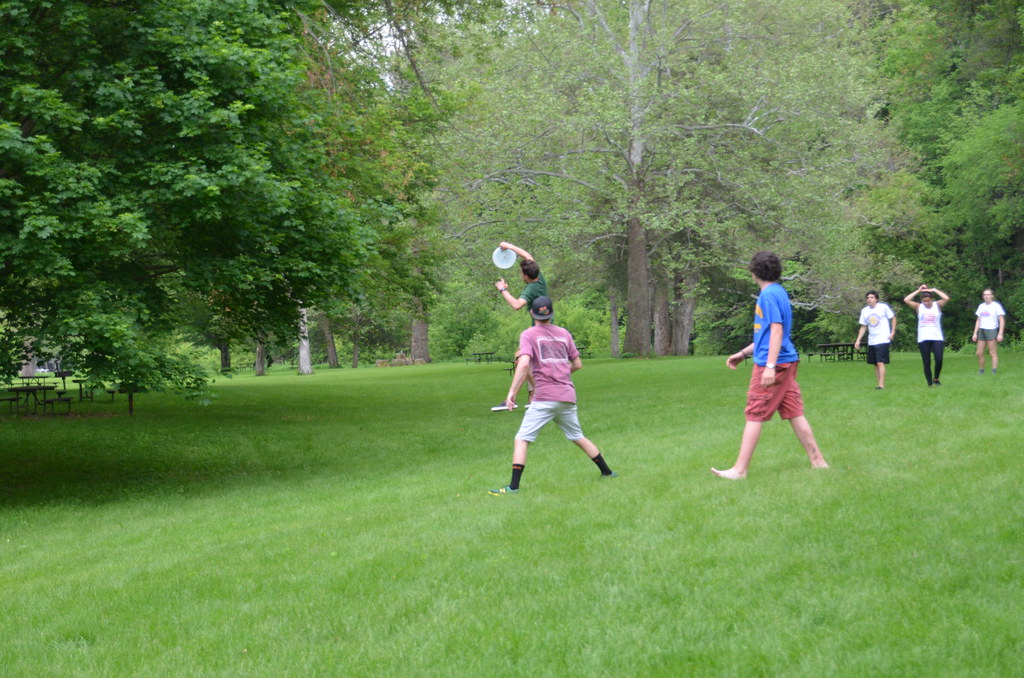In a large, lush, green park on an overcast day, six young individuals — five boys and one girl — are engaged in an animated game of frisbee. Dominating the scene, a tall boy in a green t-shirt leaps high, likely having just caught the frisbee amid shouts of excitement. Right behind him stands another boy in a magenta t-shirt, gray shorts, high black socks, and green and yellow New Balance sneakers. At the forefront, another barefoot player, donned in a blue t-shirt with yellow writing and red shorts, positions himself ready for action. In the background, the girl, wearing leggings and a tank top, ties her hair up into a bun. Two more boys in white t-shirts, one with black shorts and the other with green shorts, focus intently on the game. Mature trees, varying from fully-leaved to sparse, form a serene natural backdrop, encapsulating the energetic spirit of this friendly competition.